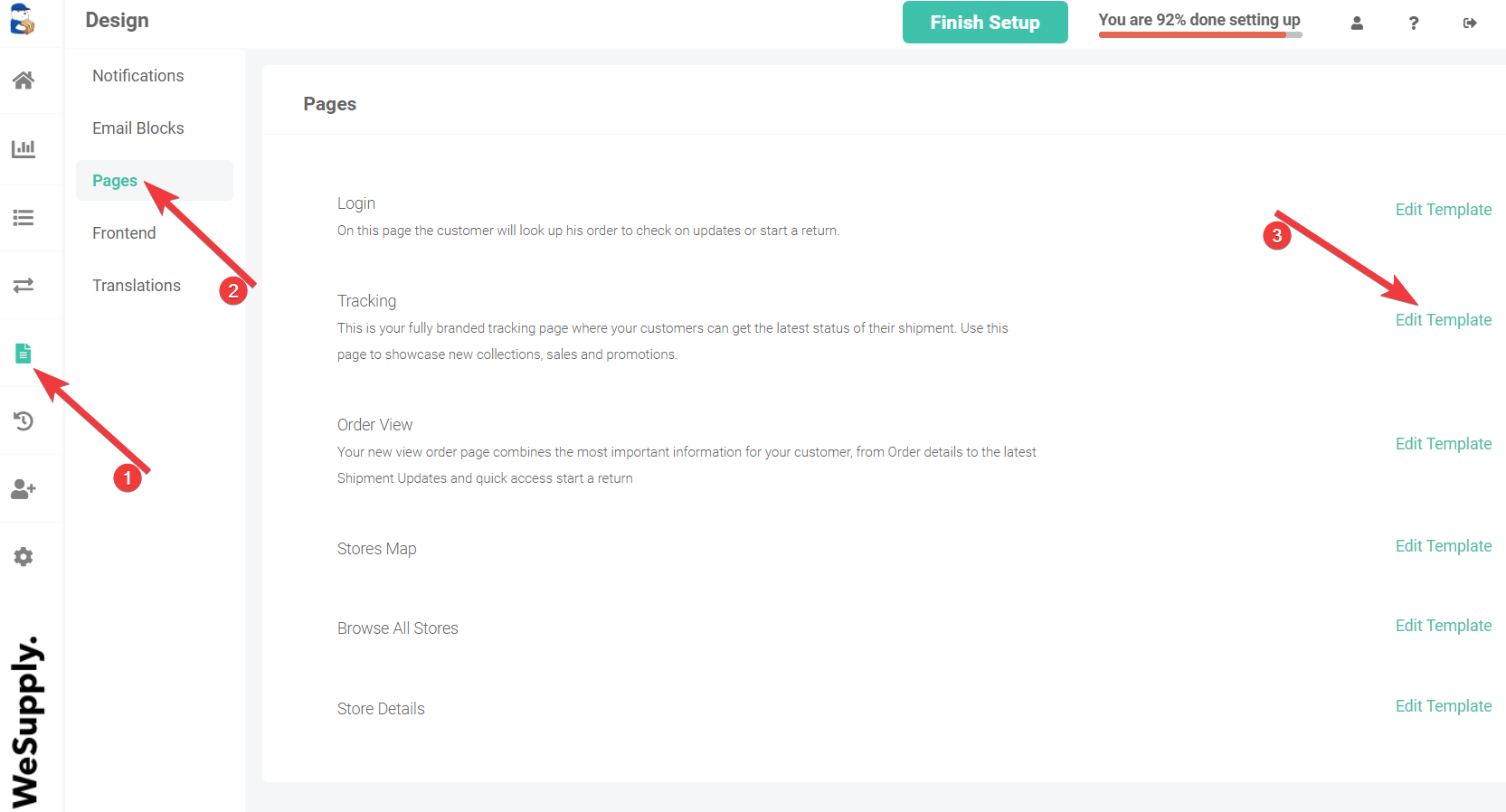The image features a stark white backdrop, serving as a blank canvas for the main elements on the screen. Positioned on the left side is a vertical menu bar, prominently displaying the company name "WeSupply." The name is presented in bold typeface with a period at the end, and it is rotated 90 degrees counterclockwise for a distinctive vertical layout.

Above the company name, there are several icons aligned vertically. Starting from the top, the icons are as follows:
1. A gray gear icon, likely representing settings.
2. A gray "add person" icon for user addition.
3. A gray undo button for reverting actions.
4. A light green (teal) document icon for managing documents.
5. Gray right and left arrows for navigation.
6. A gray bullet list icon.
7. A gray page layout icon.
8. A gray home icon, symbolizing the home page.

To the right of the vertical menu bar, a series of menu items are listed horizontally: "Notifications," "Email Blocks," "Page," "Front End," and "Translations." This setup suggests a user interface geared towards content management, providing access to various administrative functions and customization options.